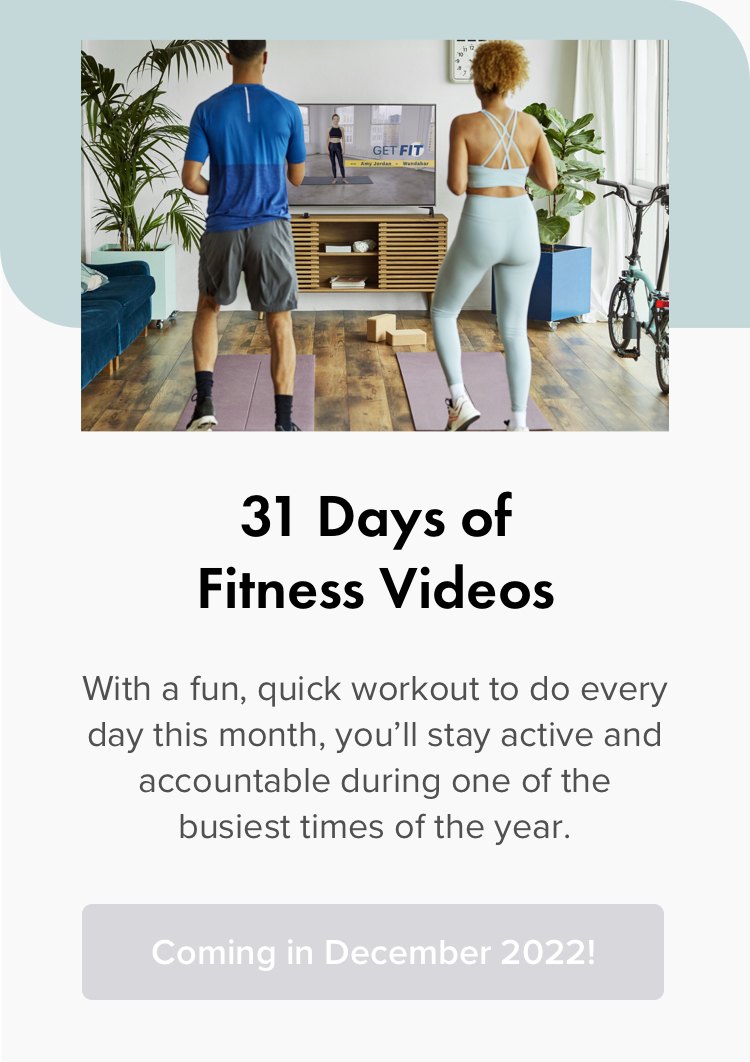A group of people stands in front of a TV screen displaying what appears to be a fitness video, reminiscent of Wii Fit, highlighting a vibrant "31 Days of Fitness" challenge. They are looking directly at the viewer, exuding motivation. Below the video, text encourages daily commitment to fitness throughout the busy month, ensuring accountability. The key information is accentuated in green and gray, with a light gray box announcing "Coming in December 2022!" against a slightly darker background. This image is part of an app announcement focused on promoting a consistent fitness routine during one of the busiest times of the year.